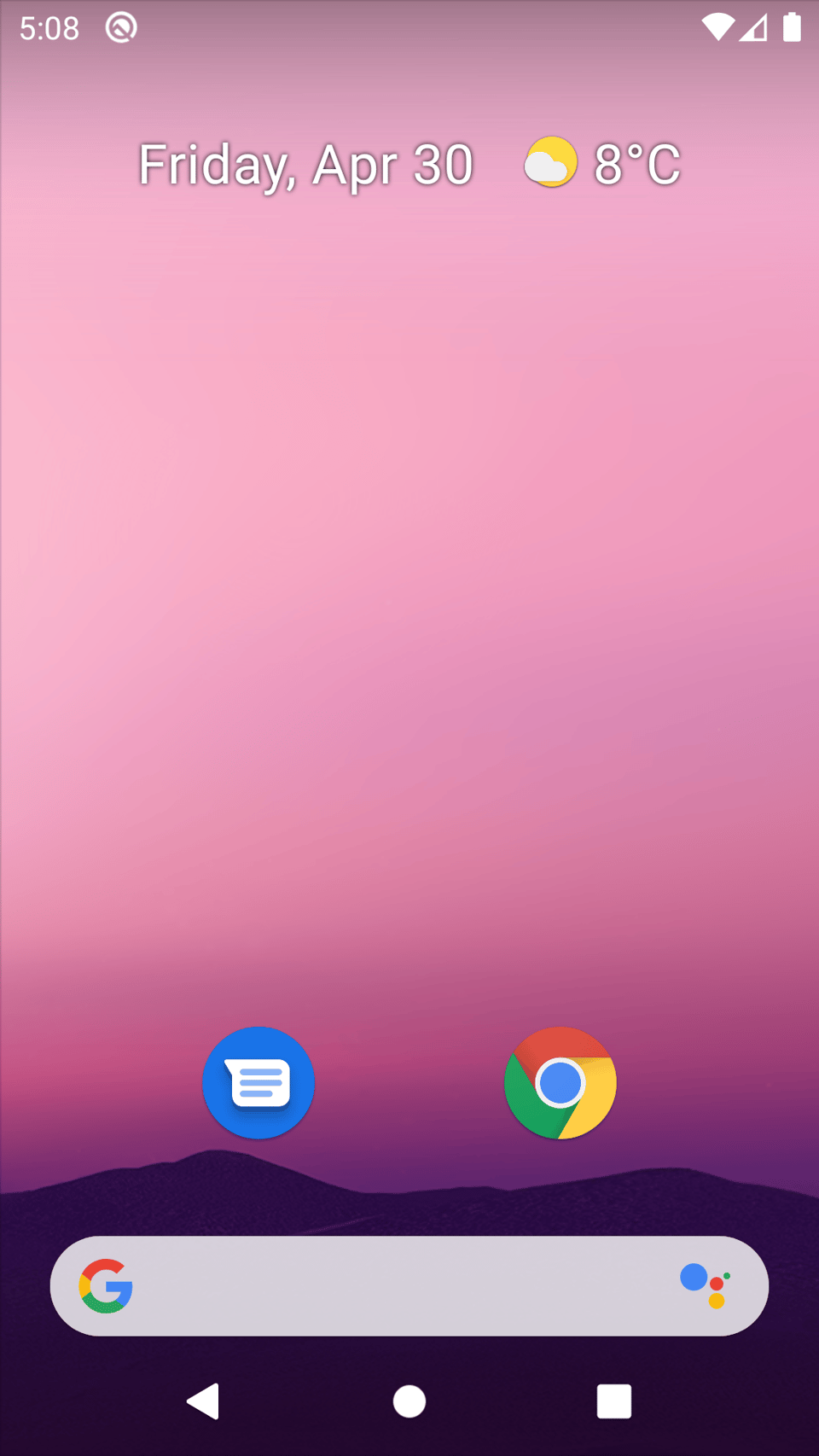This image is a detailed screenshot of a cell phone's main home screen. At the top, the time is displayed as 5:08. To the right of the time, there is a circular icon with a break and a white figure inside it, whose function is unclear. Following this, there is a Wi-Fi icon that appears like a piece of pie, indicating an active Wi-Fi connection. To its right, a triangle with two out of five bars indicates the phone's cellular signal strength. Further right, a fully white battery icon shows 100% charge.

Beneath these status indicators, the date is displayed as "Friday, APR 30," clearly indicating it is the 30th of April on a Friday. Adjacent to this date, a weather icon shows a yellow circle with a cloud, indicating fair weather conditions and a temperature of 8 degrees Celsius.

The main portion of the screen features two apps. On the left, a rounded blue app icon with a thinking or text bubble, representing the messaging application. To its right is the Google Search app icon. Below these apps is a gray search bar featuring the Google "G" logo on the left and several multicolored dots on the right.

At the very bottom of the screen, white icons for navigation include a triangle (Back), a circle (Home), and a square (Recent Apps). The entire background showcases a mauve-colored sunset or sunrise that transitions from lighter hues at the top to darker shades at the bottom, with the lower 20% of the screen depicting black silhouettes of foothills or mountains.